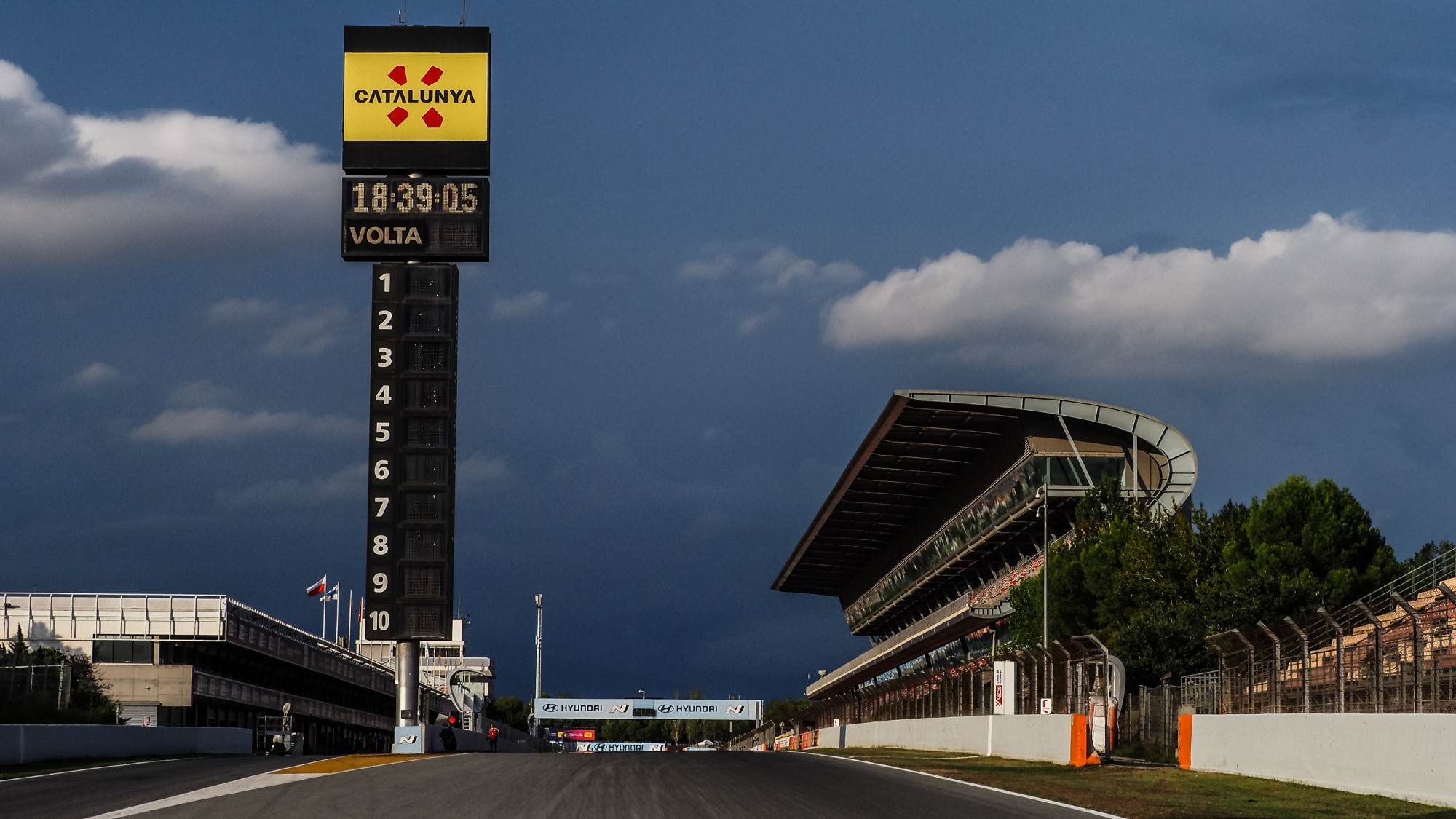The image captures a rectangular outdoor scene that appears to be a drag strip, photographed from the center of the asphalt. Dominating the scene is a towering sign, about 30 feet high, with a black board sectioned into distinct parts. The topmost section of the sign is yellow with the word "Catalunya" printed in white letters, encircled by four red X-shaped markings. Directly below this is another black section displaying the numbers "183905" followed by the word "Volta." Beneath this are vertically arranged white numbers ranging from 1 to 10.

To the right of the image, there are spectator stands, featuring a structure resembling an extended backward 'C'. The back of the scene shows the starting line of the strip, with multiple "Hyundai" banners. On the left, there is a white wall with orange ends, a possible skybox or seating building, and additional structures in the distance. The sky is depicted as a dark blue with heavy clouds, suggesting an imminent rain, and the overall atmosphere hints at a late afternoon setting.